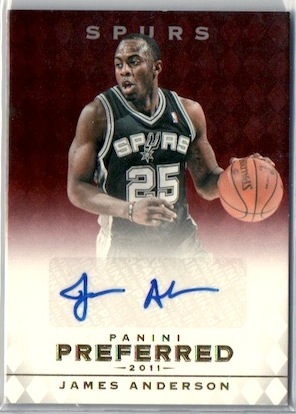This image is of a sports trading card featuring James Anderson from the San Antonio Spurs, primarily highlighting an action shot of the player. James Anderson, a 30-ish black man, is depicted in motion, dribbling a basketball with his left hand and looking to his right, his mouth open, possibly mid-play. He is wearing the black and white Spurs jersey with the number 25. The background of the card transitions from a dark red at the top to a light red, then pink, and finally white near the bottom. An authentic blue signature, which seems to begin with "J" and "A," is just below his photograph, indicating that it was personally signed by James Anderson. Below the signature, the card displays "Panini Preferred 2011" in gold lettering, accompanied by a horizontal gold bar, and his name "JAMES ANDERSON" in smaller gold capital letters. The words “Spurs” and other team details are prominently displayed at the top, emphasizing the team affiliation. The card appears to be sealed in plastic, indicating it may be a collector's item.